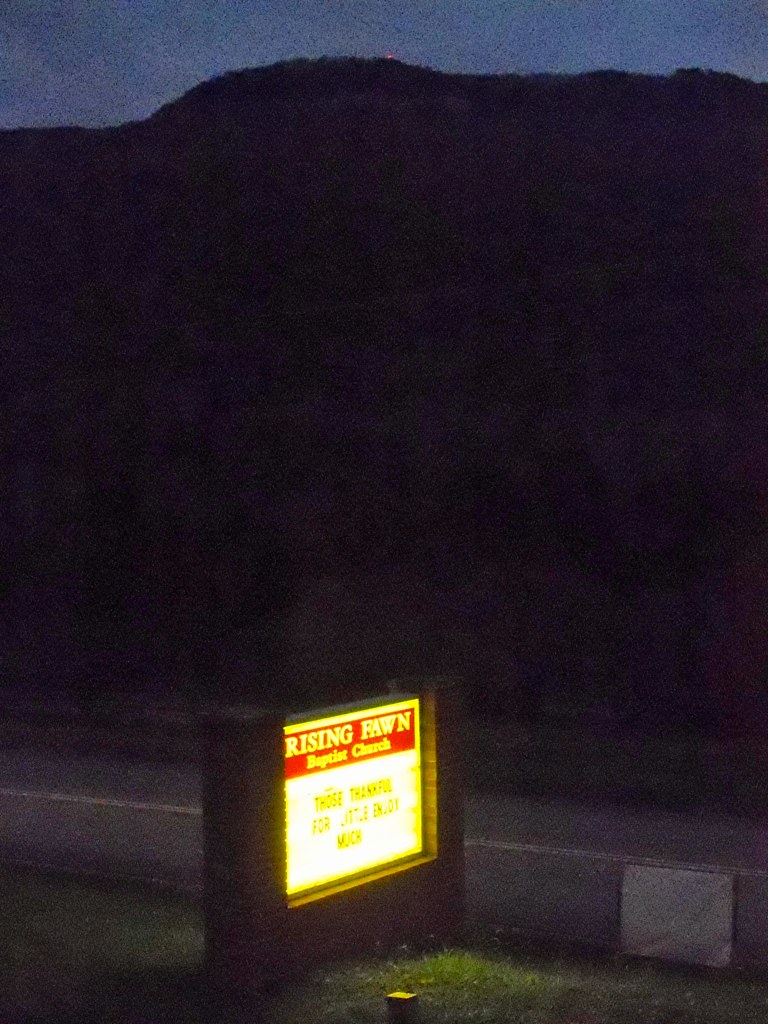This color photograph captures a serene night scene. At the top, a fragment of the deep blue night sky peeks through, suggesting the onset of dusk. Below the sky, a dark silhouette of a mountain range or hill looms, shrouded in darkness. The lower portion of the image features a grey road marked by a thin white centerline, cutting across the scene horizontally. On either side of the road, patches of grass are faintly illuminated.

The central focus of the image is a squarish sign that emits a soft glow, bordered by a black band. This sign casts light on a small yellow leaf at the bottom and a rectangular grey object situated towards the bottom right corner of the picture, both bathed in a white and yellowish light. The sign itself has a red rectangular section at the top adorned with unreadable yellow text, possibly advertising or indicating something. Below this, the sign features a white section with additional yellow writing that remains indecipherable. The interplay of light and shadow creates a tranquil yet mysterious atmosphere.